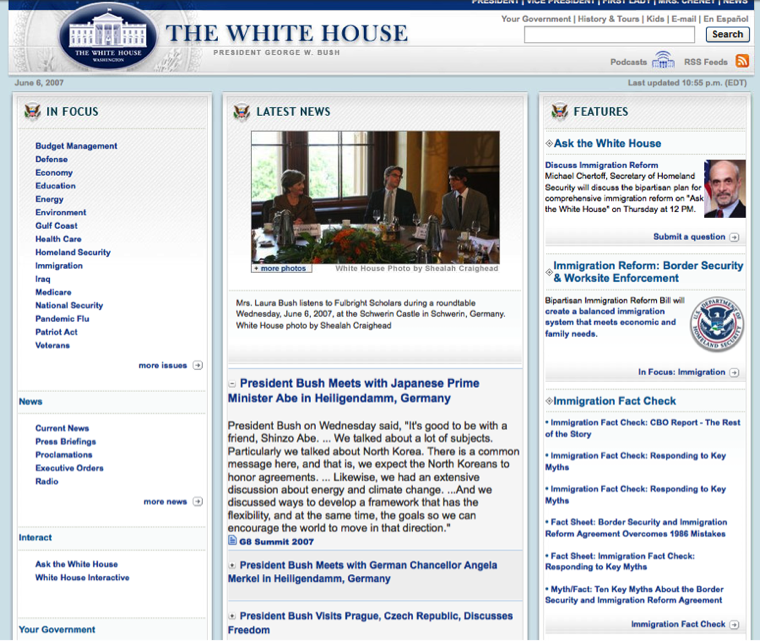The screenshot features the homepage of the White House website during President George W. Bush's administration, dated June 6, 2007. The site organizes information into several key categories, including budget management, defense, economy, education, energy, environment, Gulf Coast recovery, healthcare, homeland security, immigration, Iraq, Medicare, national security, pandemic flu, the Patriot Act, and veterans' affairs, with an option to explore more issues.

A prominent section, titled "Latest News," includes a White House photo by Sheila Craighead depicting Mrs. Laura Bush engaging with Fulbright scholars during a roundtable discussion at Schwerin Castle in Germany. Adjacent to this is news of President Bush meeting Japanese Prime Minister Shinzo Abe in Heiligendamm, Germany. The update highlights Bush's statements about their discussions on North Korea, energy, and climate change.

Additionally, the site emphasizes President Bush's attendance at the G8 Summit 2007 in Germany and his meetings with German Chancellor Angela Merkel and visits to Prague in the Czech Republic. An article under "Featured" invites users to join an "Ask the White House" session about immigration reform, noting that Michael Chertoff, Secretary of Homeland Security, will field discussions on the bipartisan immigration reform plan. This feature includes a comprehensive "Immigration Fact Check," countering common myths and providing detailed reports from the CBO.

The detailed, user-friendly layout offers numerous interactive elements, such as the ability to ask questions directly to the White House or read more factual updates on recent legislative efforts and governmental policies.